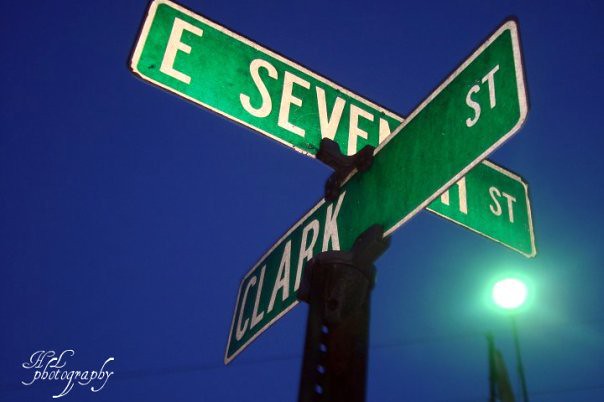In the bottom left corner of the image, the words "HL Photography" are elegantly inscribed in white cursive script. The scene is set towards dusk or evening, as indicated by the dark blue hue of the sky, almost transitioning into nighttime. On the right side of the picture, a lamppost is visible, casting a warm glow as its light is turned on. Dominating the foreground is a street sign at an intersection, featuring two distinct signs with a common design. The lower sign prominently displays "Clark" in large, bold white letters on the left side, followed by "ST" for street on the right side, all against a green background with a white border. The upper sign, also with a white border and green background, reads "E 7th" on the left side, though the "TH" in "7TH" is partially obscured. To the right of "E 7th," it again reads "ST" indicating street.